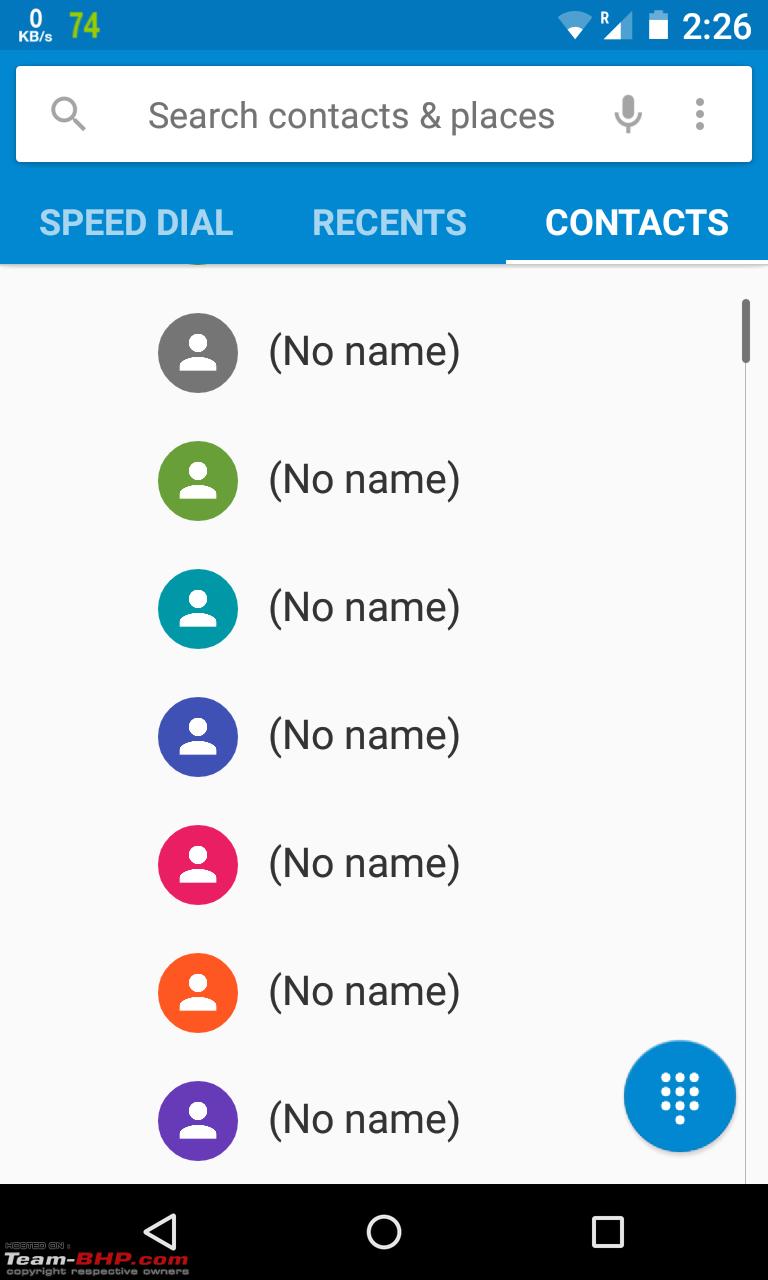This is a screenshot of a person’s phone interface, with a visible watermark in the bottom left-hand corner indicating that it is hosted on team-bhp.com, with copyright noted as respective owners. The watermark's text is color-coded: "hosted" is in black outlined in white, "team" and the dash are in white, "bhp.com" is in red, and "copyright respective owners" appears in white against a black background that also shows the phone's navigation options.

The main section of the screen displays a contacts list against a white background, with each contact labeled as "No Name." To the left of each "No Name" entry, there are colorful icons depicting a generic person’s bust. On the right side of this section, a circular icon for accessing the dial pad to input phone numbers is visible.

At the top of the screen, a blue box houses a white search bar labeled "Search contacts and places." Below this search bar, still within the blue box, are options for "Speed dial," "Recents," and "Contacts," with "Contacts" currently selected. 

The very top part of the screenshot shows the phone’s status bar, displaying essential information such as the battery percentage, Wi-Fi connection status, signal reception strength, and the current time.